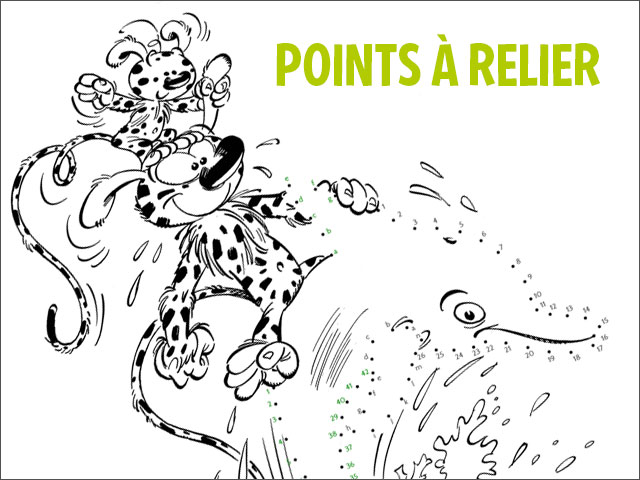The image is a page from a children's coloring book that depicts a whimsical scene combining elements of a connect-the-dots puzzle and cartoon art. The main illustration, rendered primarily in black and white with some red accents, features two humorous, cat-like animals with exaggerated features, such as large ears, cartoon eyes, and long, spotted tails that are twice the length of their bodies. One animal stands on the head of the other, with both characters exhibiting a playful, smiling demeanor. The lower animal appears to be riding a dolphin that bursts out of the water, complete with splashes at the base. However, the dolphin's outline is incomplete, as it is designed to be finished by connecting the numbered dots. The upper right corner of the page contains text in medium green letters, reading "points are relier." Some dots in the dot-to-dot puzzle are highlighted in green and red, adding to the interactive and colorful nature of the activity.